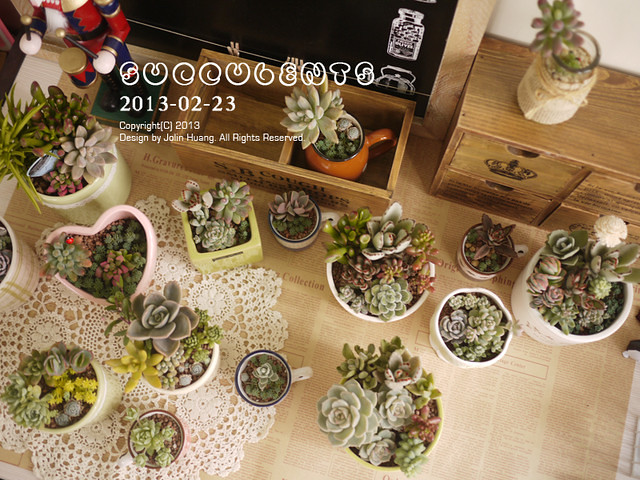In this bright, top-down photo taken on February 23rd, 2013, designed by Jolin Huang, we see an artistic arrangement of various colorful succulents. The succulents, which come in shades of green, purple, and light lilac, are planted in an assortment of containers including coffee cups, small bowls, and planters of different shapes and sizes. Some planters are round, while one noted is square and green. There are six planters arranged on a white doily on the left side of the table, with additional planters positioned to the left and towards the back. Among these, there's a heart-shaped planter pot also on the doily.

A small wooden bookshelf-like structure holds one of the succulent containers, and a wooden box on the table supports a jar covered in cloth and tied with a bow. An old, faded newspaper or newsprint serves as the backdrop on the table, enhancing the vintage feel. Additionally, a nutcracker, hinting at Christmas decoration, is visible in the upper left corner. The entire scene, marked with the artist's copyright and the date, showcases a charming and varied display of succulents in an eclectic mix of planters.